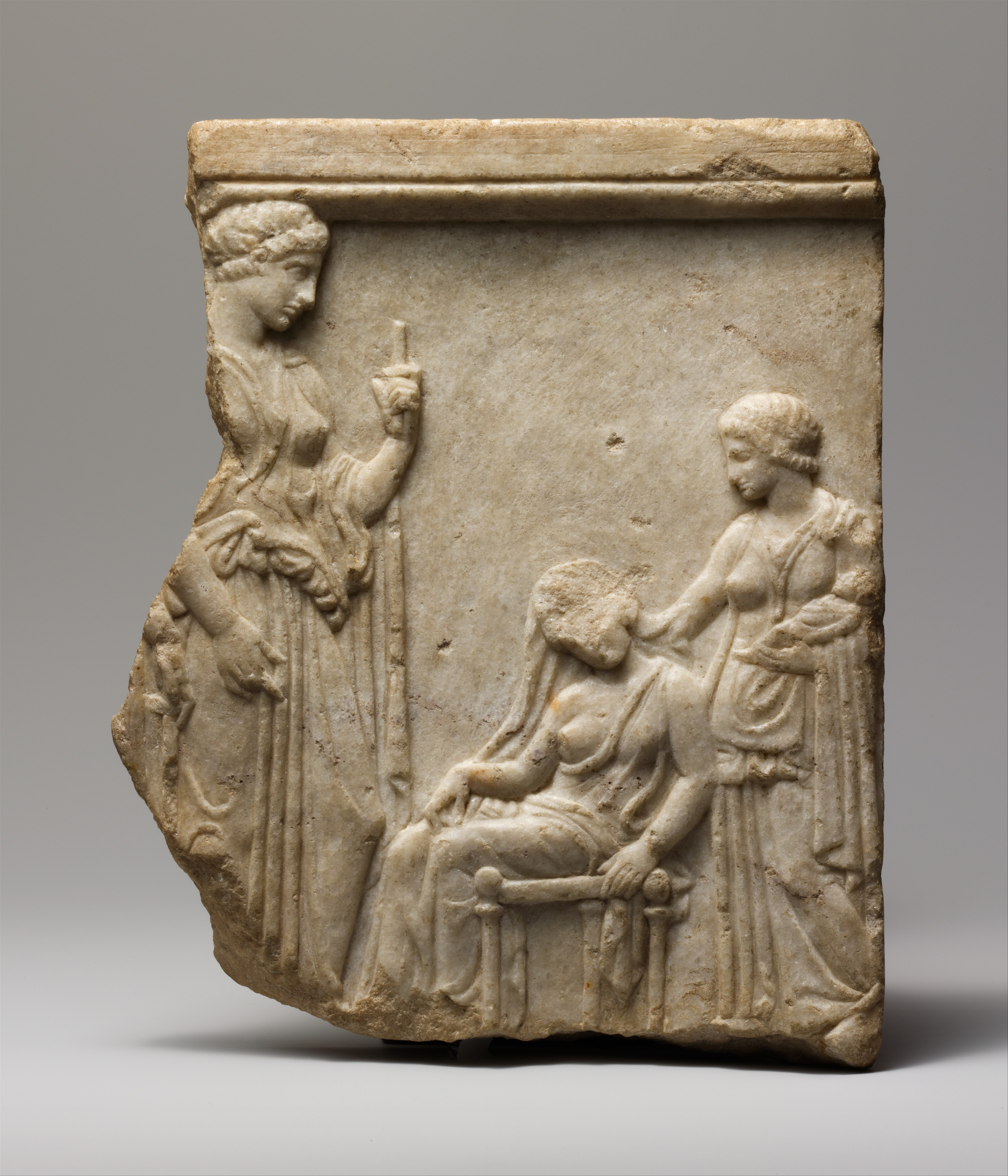The image depicts a detailed, beige-colored marble relief sculpture set against a gray background. The carving seems slightly damaged, suggesting parts may have broken off over time. Featured in the scene are three people in outdated clothing that resembles robes. On the left, a prominent woman with curly hair tied up in a bun and a dress that flares outward stands gazing to the right. Her raised arm appears broken at the elbow, indicating possible damage. In the center, a seated figure has hair obscuring their face and appears slumped, conveying a sense of weariness or injury. To the right, another woman with her hair pulled back tends to the seated figure, suggesting she is possibly arranging their hair. This intricate carving, adorned with a top border, carries an air of solemnity and historical significance through its detailed and expressive depiction of the figures.